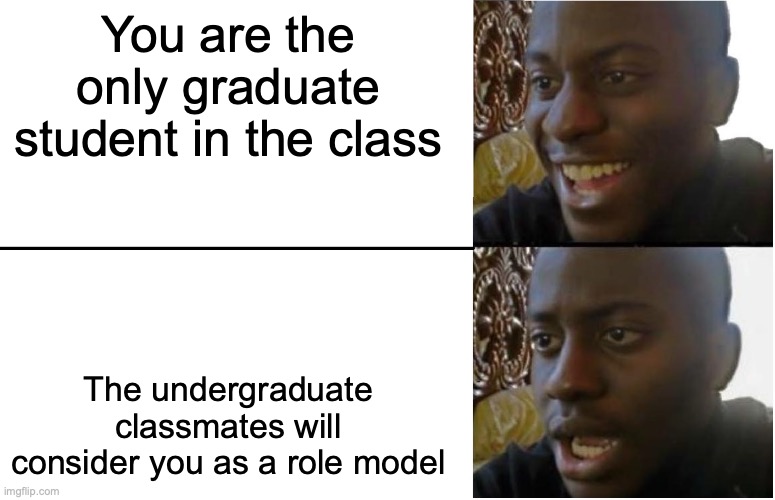This meme features two side-by-side images of a young Black man wearing a black hoodie, set against a background with a mix of brown, white, and yellow. The image is divided horizontally with a black line. 

In the top image, the man's face shows a joyful expression, with a wide smile and bright eyes. The background is a pattern combining brown, white, and yellow on the left and plain white on the right. The text next to this image, set on a stark white background with black letters, reads: "You are the only graduate student in the class."

In the bottom image, the man's demeanor changes to one of disappointment, with a noticeable absence of a smile and a somewhat dimmed look in his eyes. Again, the background remains divided into patterned and plain sections. The accompanying text to this image states: "The undergraduate classmates will consider you as a role model." The bottom left corner of both images bears the watermark "imgflip.com." Additionally, in the lower image, the man's chin is slightly cropped out. 

The meme juxtaposes the initial pride and subsequent pressure felt by the graduate student upon realizing the expectations placed by his undergraduate peers.